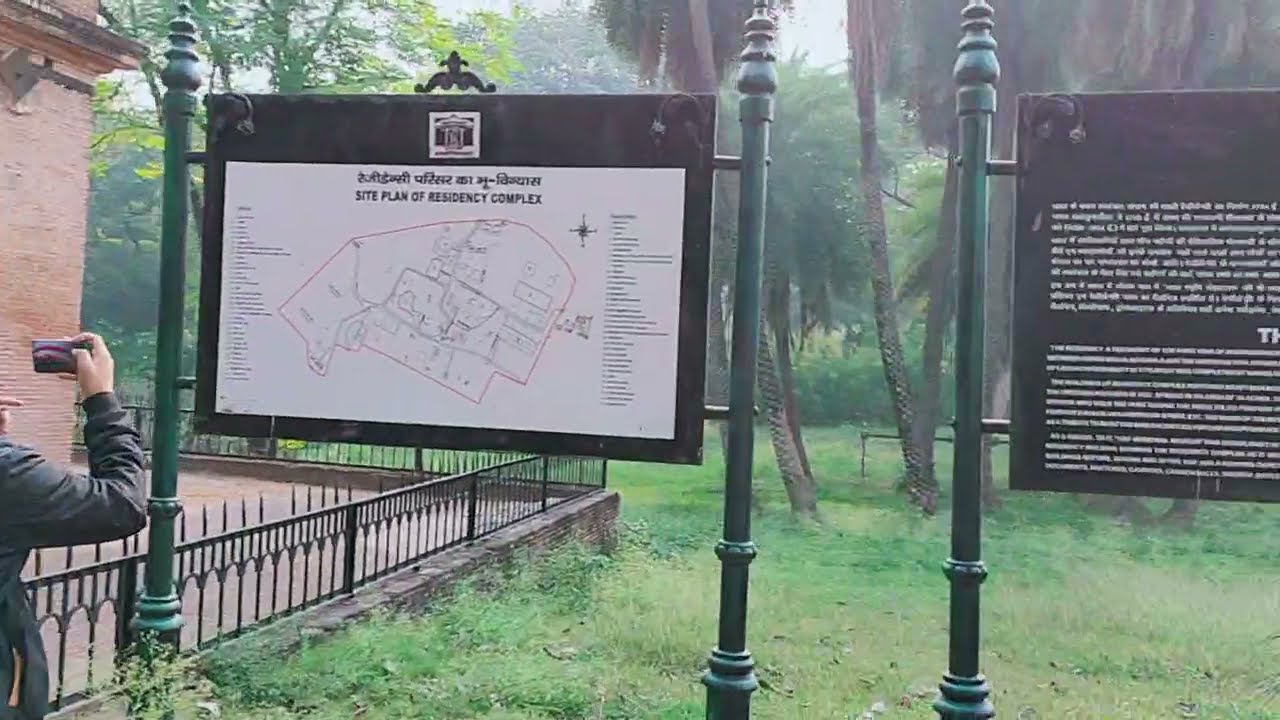The image depicts an outdoor scene that appears to be an entrance to a park or a residential complex. In the foreground, there are two black signs posted on green poles. The sign on the left features a site plan describing a "Residency Complex," highlighted with black text including some non-English lettering at the top, and a detailed layout outlined in red. The sign on the right has a black background with tiny white font that's difficult to read, supported by a single green pole visible in the image. To the left of these signs stands a brick building, partially obscured by a low half-black fence. A person wearing a long black jacket is seen extending an arm to take a picture with a smartphone. The background is filled with lush green grass, several large trees including palm trees, and dense leafy vegetation, suggesting a well-maintained outdoor space. The overall ambiance indicates it could be either spring or early fall.